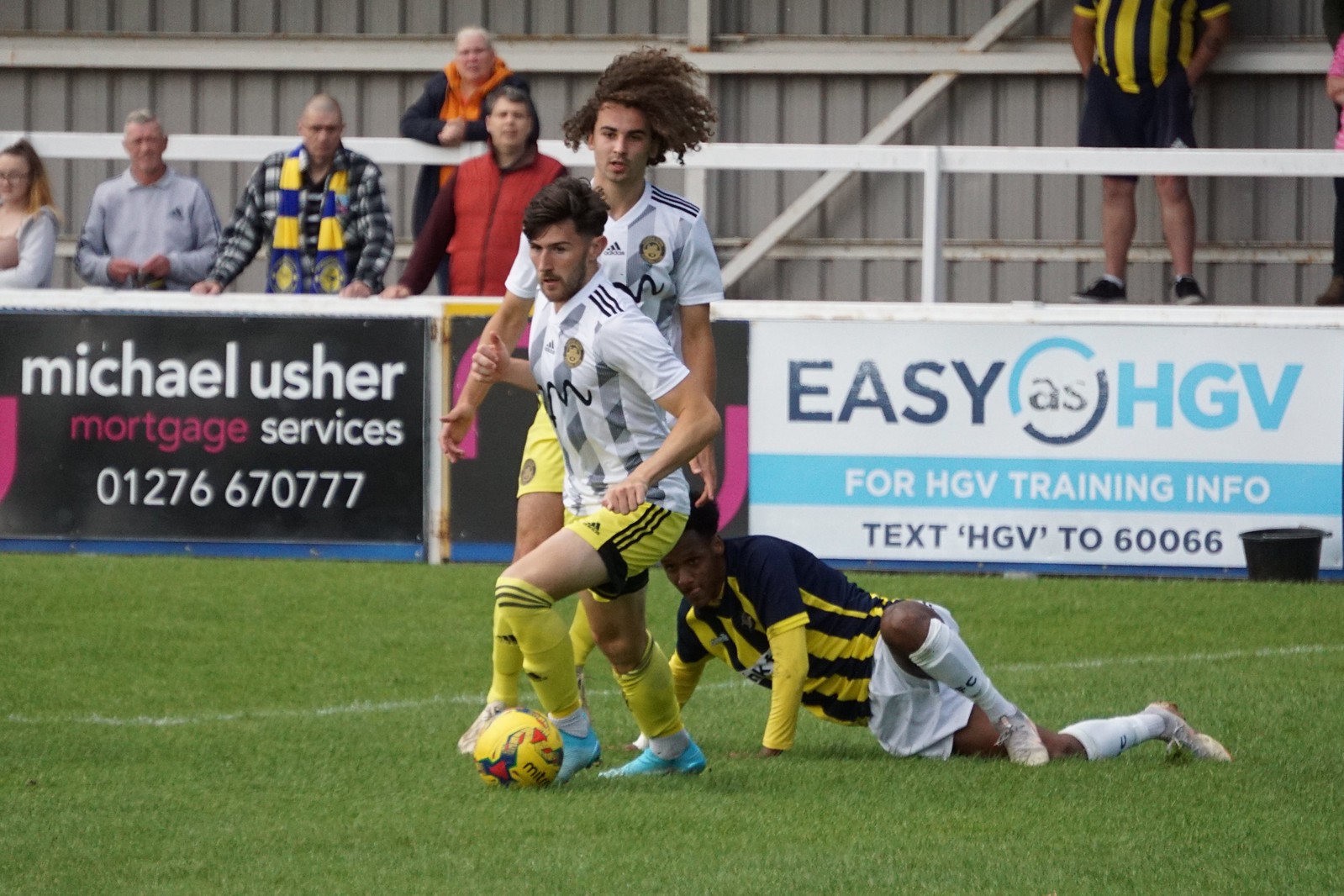The photograph captures a lively moment in an English soccer match, featuring three players on a grassy field with relatively empty stands behind them. Prominent in the scene is a player dressed in a dark blue jersey with yellow stripes and white shorts who has fallen to the ground. Ahead of him are two players in white jerseys with yellow and black shorts, one of whom is poised to kick a yellow soccer ball. The backdrop includes several advertisement panels with logos such as "Easy as H-U-G-V" and "Michael Usher Mortgage Services," and a noticeable, albeit sparse crowd. The left side of the stands shows about five spectators intently watching the unfolding action, while a few more on the right are partially visible, standing and observing from their vantage points.